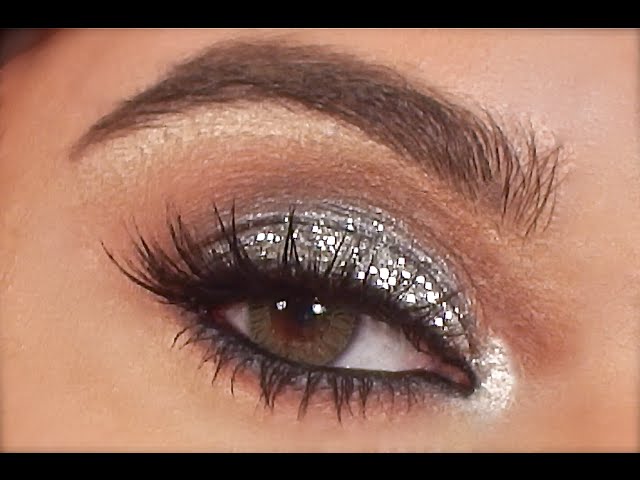The image appears to be a screenshot from digital media, with noticeable black borders on the top and bottom. It prominently features a close-up of a female eye, adorned with elaborate makeup. The eyelids are covered in silver glittery eyeshadow that shimmers, possibly reflecting light from the sun or studio lighting. The eyelashes, heavily coated with mascara, are long and might be enhanced with falsies. The skin around the eye has been meticulously touched up and has a pinkish hue, with blue eyeliner accentuating the lower lid. The eyebrow is carefully groomed, arching above the eye—starting lower on the right side, peaking towards the top, and descending slightly on the left. The eye itself is a captivating greenish-brown, with a large pupil ringed in brown, giving it a striking appearance. The image is slightly pixelated, hinting that it could either be a video screenshot or a low-resolution photo.